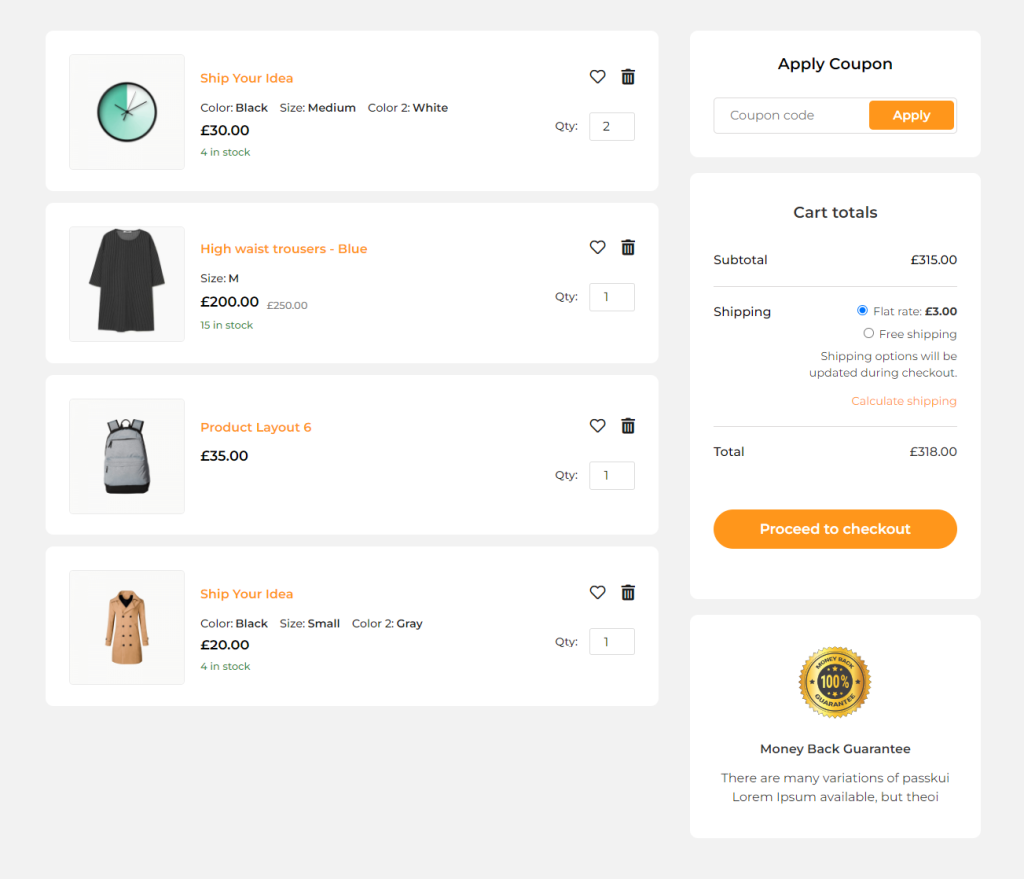The image is a screenshot of an online shopping cart from a website. The cart lists several items with detailed descriptions and pricing information as follows:

1. The first item is titled "Ship Your Idea." It is available in two colors and sizes:
   - Color: Black, Size: Medium 
   - Color 2: White 
   The price for this item is £30.

2. The second item is "High-Waist Trousers," priced at £200.

3. The third item, labelled as "Product Layout 6," appears to be a backpack and is marked at £35.

4. The fourth item is another "Ship Your Idea," which seems to be a trench coat. It is described with:
   - Color: Black, Size: Small 
   - Color 2: Gray 
   This item is priced at £20.

The total cost for all items in the cart amounts to £318, and there is an additional shipping charge of $3.